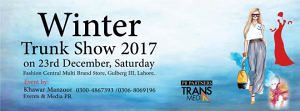This image is an advertisement for the Winter Trunk Show 2017, scheduled for the 23rd of December, Saturday. The background is blue, with the event details written in prominent black letters. To the right, the image features a collage of fashionable women. One woman is depicted holding a yellow and black bag while wearing high-waisted gray slacks, a white shirt, and sunglasses. Next to her, there is another image of a woman in a striking long red gown and a red turban. In the far right-hand corner, although slightly obscured, there appears to be someone kneeling in a red puffer jacket. The overall layout is a long, horizontal rectangular shape. The left side of the advertisement holds additional details, including an address, phone number, and possibly other less clearly defined text elements. The word "Transmed" is also visible next to the images of the women, indicating a potential sponsor or associated brand.